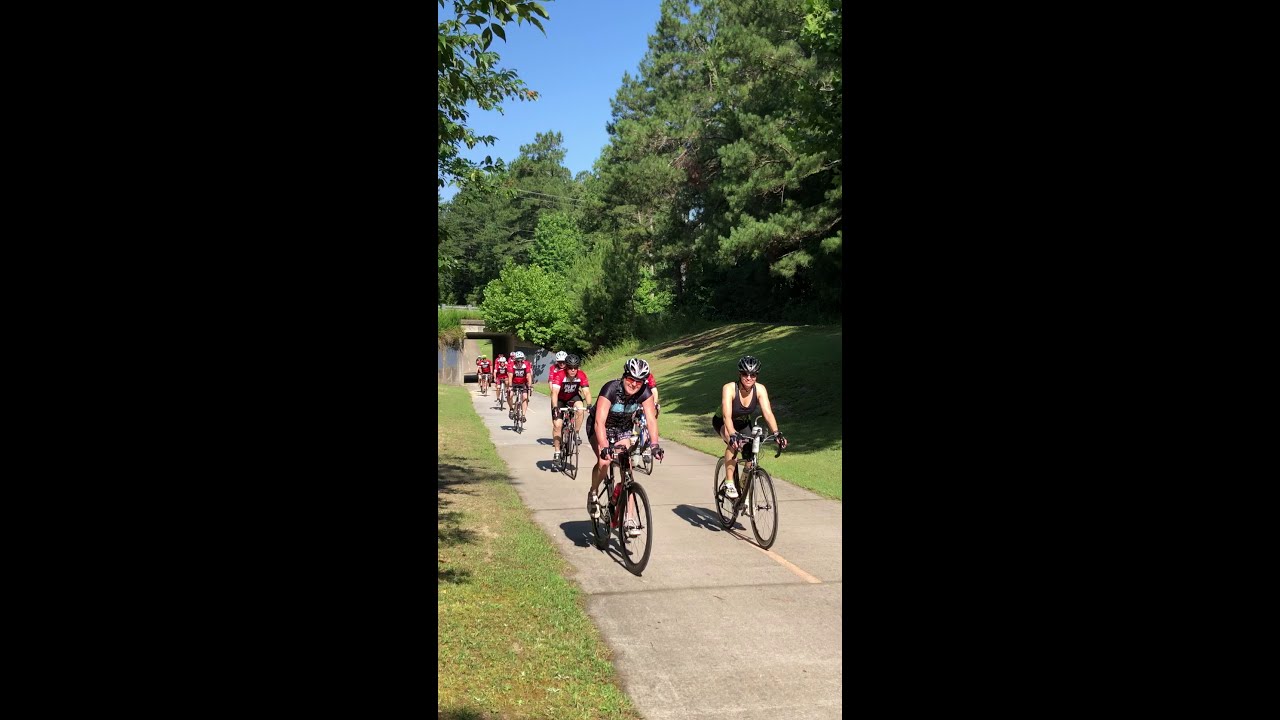The photograph captures a small group of approximately 12 bicyclists riding along a scenic, narrow bike path that winds through a well-manicured park. The setting is bright and sunny, accentuating the verdant greenery and well-maintained grass that flank the path. The trail, which seems more like a paved pathway than a road, stretches into the distance, where it passes under an overpass nestled among lush trees and bushes. 

In the foreground, the lead cyclists—a man and a woman—are dressed in black clothing, contrasting with the rest of the group behind them, who wear coordinated red jerseys with black chest lettering or numbers. All riders are equipped with helmets and sunglasses, suggesting a serious, perhaps competitive cycling session or event. To the left in the background, a small lake or body of water glimmers subtly, adding to the picturesque quality of the scene. The vertical format of the photo focuses on the cyclists, while the left and right borders are marked by black bars, emphasizing the central activity.